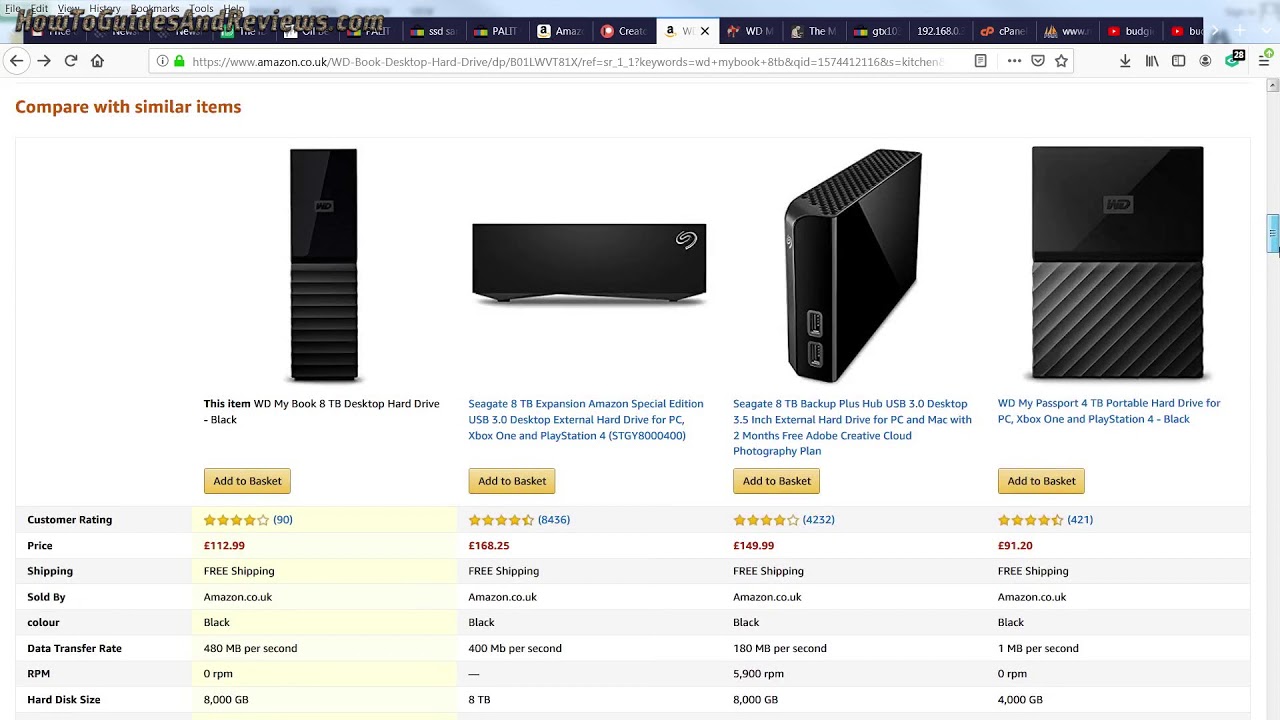The image illustrates a detailed comparison of the same speaker model from various manufacturers. It presents four different brands, highlighting aspects such as customer reviews, shipping details, and the respective manufacturers. Each option includes precise information on how it is shipped, where it ships from, and who manufactures it, aiding consumers in making an informed decision. Despite the image being somewhat blurred, one can still discern small annotations below each speaker description. Additionally, the speaker depicted has multiple tabs open on a digital interface, likely providing further detailed specifications and comparisons.